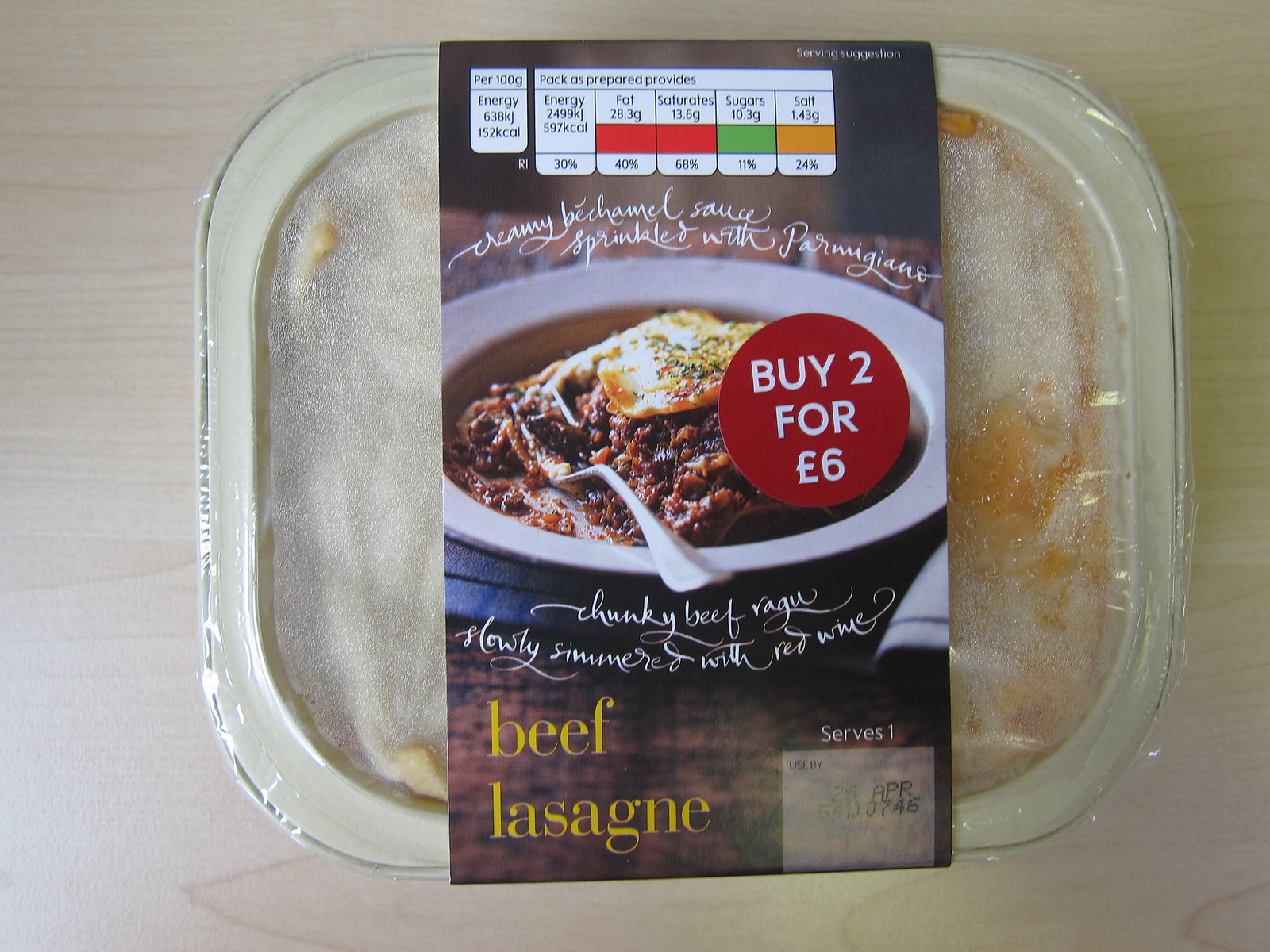A refrigerated or frozen meal labeled "Beef Lasagna" sits on an almost white, light brown table. The packaging features a black and white bowl filled with beef lasagna, prominently showcased. At the bottom of the packaging, "Beef Lasagna" is written in yellow. Above this text, the image of the lasagna is accompanied by a concise description: "Chunky beef ragu slowly simmered with red wine." Above the bowl, it reads, "Creamy béchamel sauce sprinkled with Parmigiano."

To the side, a red circle with white text announces a promotional offer: "Buy two for £6." At the top of the packaging, the nutritional information is clearly listed per 100 grams. It details the energy content as 638 kilojoules and 152 Kcal, with 28.3 grams of fat, 13.6 grams of saturates, 10.3 grams of sugars, and 1.43 grams of salt. Beside these figures, the daily percentage values for each nutrient are provided for easy reference.